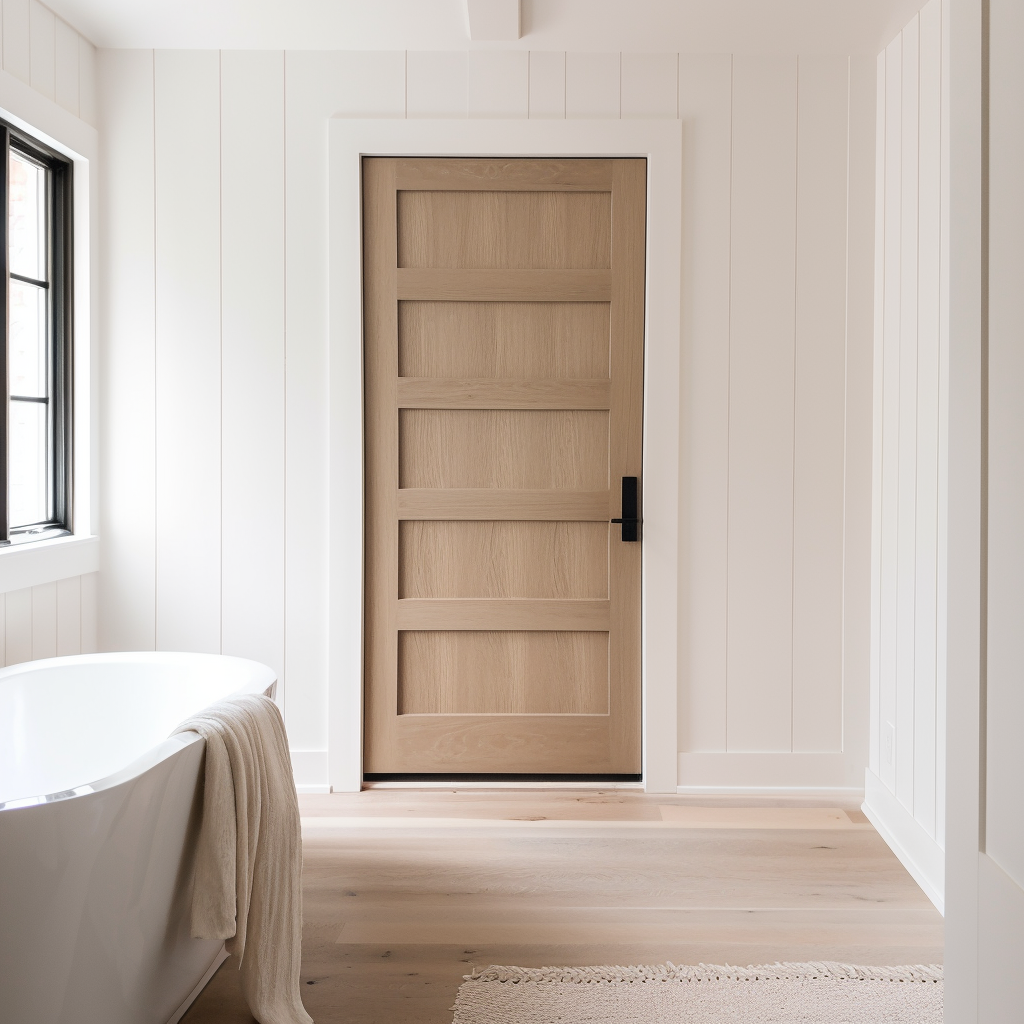This photograph captures the serene interior of a bathroom bathed in light. It features elegant light hardwood floors adorned with a small beige throw rug in the bottom right corner. Dominating the left side of the image is a pristine, stand-alone white ceramic bathtub, adorned with a towel draped over its edge. The background showcases a premium wooden door, distinct with its five horizontal panels and a sleek black doorknob. White paneled walls with vertical lines enclose the space, accentuating the simplicity and brightness of the room. A window with three slots is positioned to the left of the door, allowing natural light to enhance the airy ambiance.